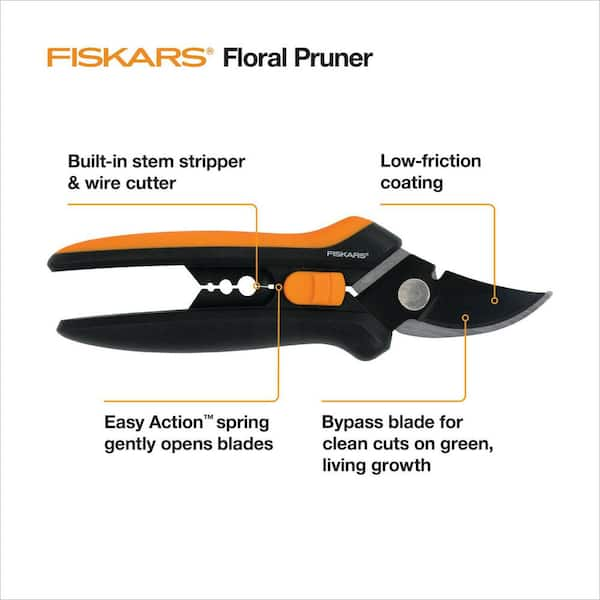The square image features a Fiskars Floral Pruner with a light gray thin border and a white background. At the top, "FISKARS®" is written in all caps in orange letters, followed by "Floral Pruner" in black. The central section of the image contains various annotations with orange lines pointing to different parts of the pruner. It highlights key features in black font such as "Built-in Stem Stripper and Wire Cutter" on the left, and "Low Friction Coating" just to the right. The pruner itself is displayed horizontally with the pointed blade end towards the right. It has an orange handle top and a black body with a silver-edged black blade. An orange sliding knob is situated in the center. At the bottom left, the text "Easy Action Spring, gently opens blades" is present with an orange line pointing upwards. In the lower right, "Bypass Blade for Clean Cuts on Green Living Growth" appears with a corresponding orange line. The wire cutter accommodates different wire sizes and the blade is designed for sharp, precise cuts.